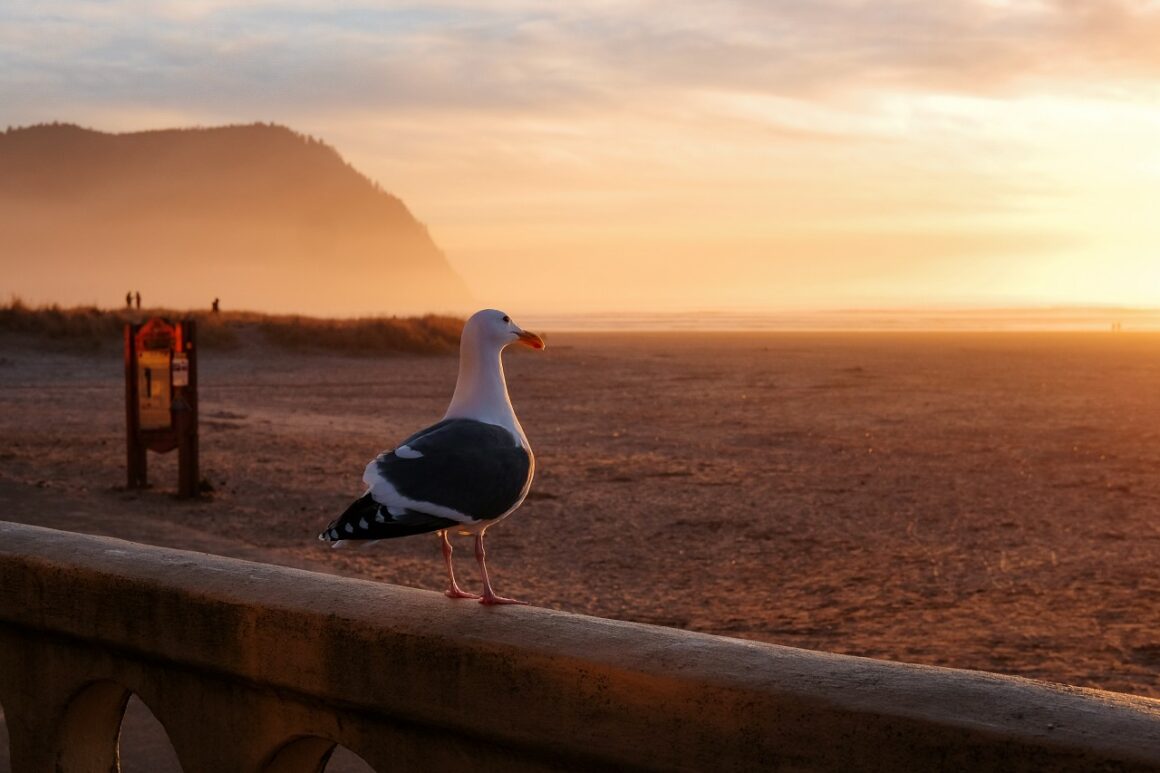This photograph captures a serene beach scene with a seagull perched on an old wooden railing, gazing out over the ocean as the sun sets. The seagull stands prominently in the center of the image, showcasing its striking features: an orange beak, white head and neck, gray body with black and white-tipped wings, webbed orange feet, and black eyes. The sky is painted in vibrant hues of orange and red, indicating that the sun is just dipping below the horizon, casting a warm glow over the scene. In the background, the tranquil water meets the edge of a wide, open beach that transitions into grassy patches. To the left of the bird, a wooden sign stands near the railing, and silhouettes of people are visible in the prairie grass, adding a sense of life and scale to the composition. Distantly, a large cliff or mountain looms, completing the picturesque coastal landscape. The overall atmosphere is one of peaceful reflection, with the seagull as a sentinel of the closing day.